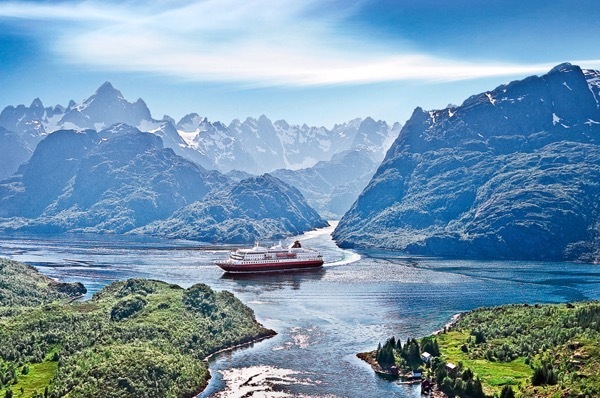This image captures a detailed and picturesque scene of a large ship, possibly a tourist or container ship, cruising through a waterway bordered by rugged, snow-capped mountains. The ship itself features striking colors, with a black hull, a red stripe, and a white superstructure dotted with numerous windows. The water takes on a cold, blue hue, and the foamy trail behind the ship indicates its swift passage.

Surrounding the waterway are dramatic mountain formations with gray rocky surfaces and patches of lingering snow, giving them a blue tinged appearance from afar. Some slopes are lush with clusters of pine trees and other greenery, contributing to the striking contrast between the verdant foreground and the more barren summits. The right side of the image features an area that might contain a small village or harbor structures.

Notably, the waterway appears to extend in all four directions, resembling a crossroads amidst the towering landscape. On the lower left and right corners, islands or peninsulas covered with green grass and tree clusters frame the ship's path. Above, the sky is a brilliant blue, hazy with elongated white clouds, enhancing the expansive feel of this dramatic and serene natural setting.